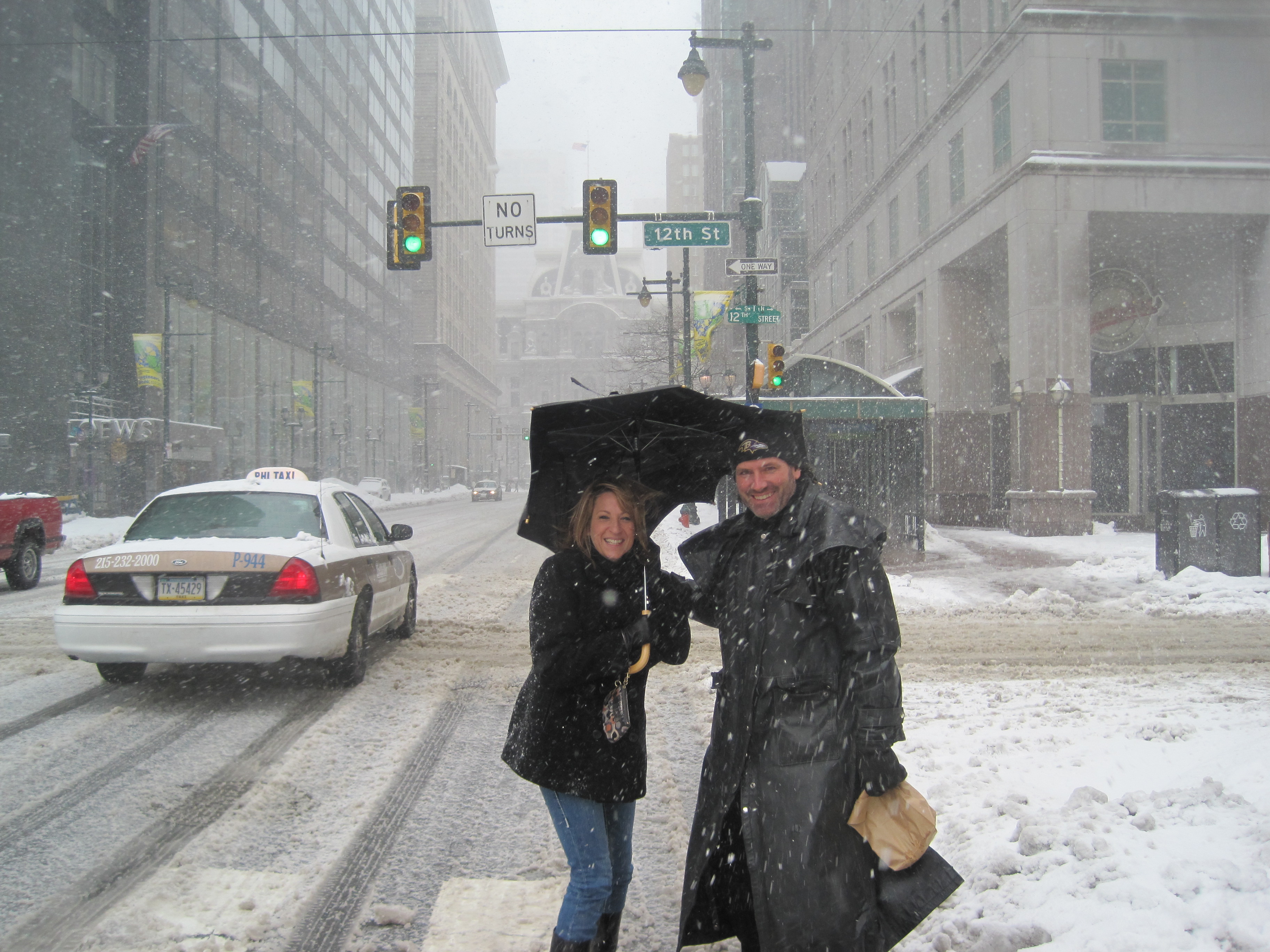In this vivid cityscape scene, two smiling individuals pose for a photograph amidst a heavy snowstorm on a bustling street corner. The man on the right is distinguished by his long black leather trench coat, black gloves, and black hat, and is holding a brown bag in his left hand. To his left, a woman dressed in a black jacket, blue jeans, and black boots stands under a black umbrella, shielding herself from the falling snow. They are surrounded by thick snow piled high on the sidewalk and tire-marked streets. Above them, traffic signals with green street signs reading "12th Street" and additional signage including a white "No Turns" sign and a one-way arrow pointing left are prominently visible. A white taxi drives away towards the left side of the image, leaving the scene marked by urban high-rises and towering buildings in the backdrop. Despite the wintry conditions, the pair radiates warmth, happily smiling at the camera.